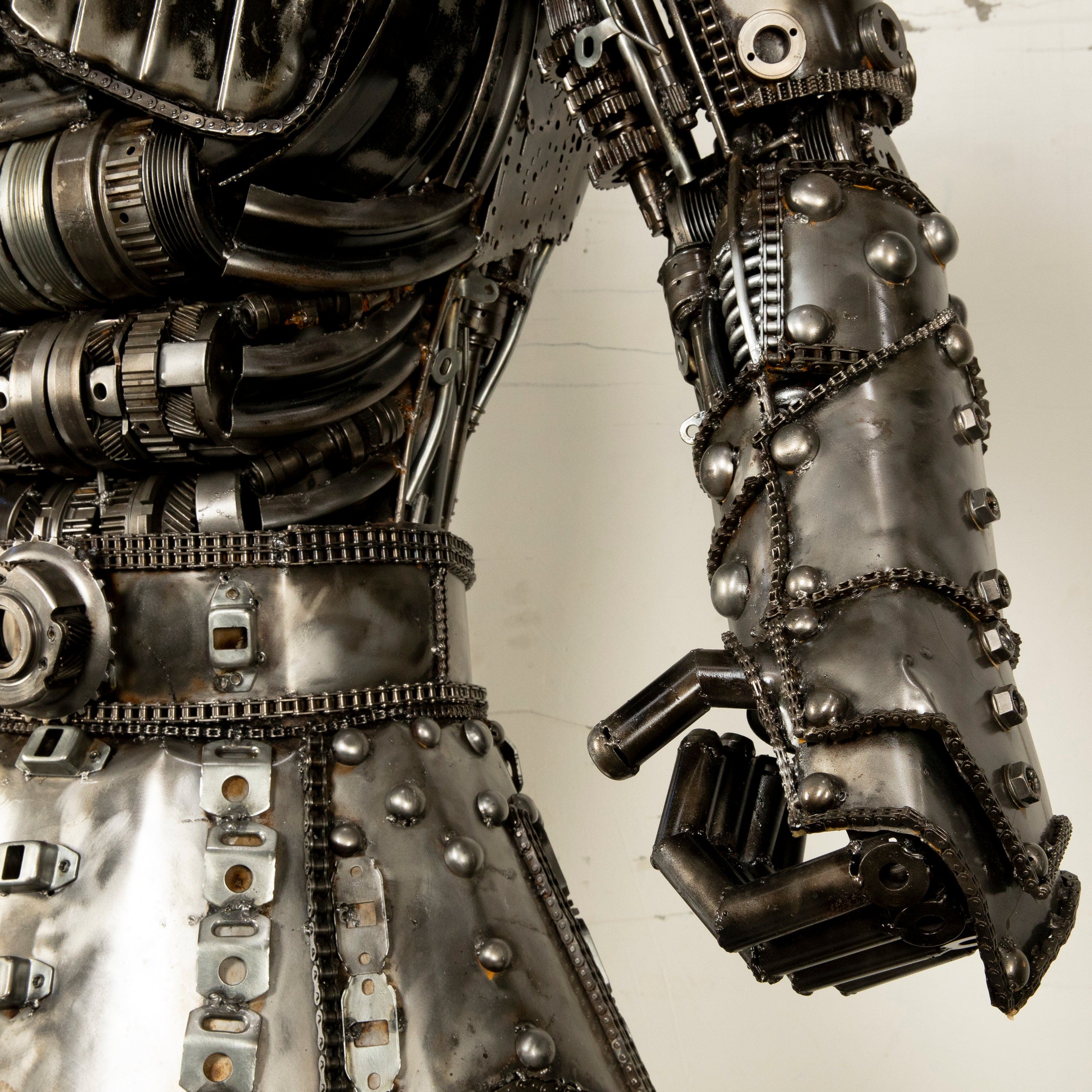The photograph showcases a detailed close-up of a steampunk-inspired, robotic armor. This elaborate design features a combination of dark and light brown metallic armor plates held together by rivets and chains. The focal point is the robotic arm, which is adorned with intricate metalwork, including a dark brown, articulated hand. The forearm and chest areas reveal additional elements such as wires, hydraulics, and steel components with a silver hue. At the center of the chest, a prominent screw secures a steel belt, and more armor plating extends downward. The entire suit exhibits numerous industrial motifs with rivets and high-quality metalwork that remains shiny and rust-free. The background highlights a cream-colored wall, emphasizing the contrast and detail of the armor.